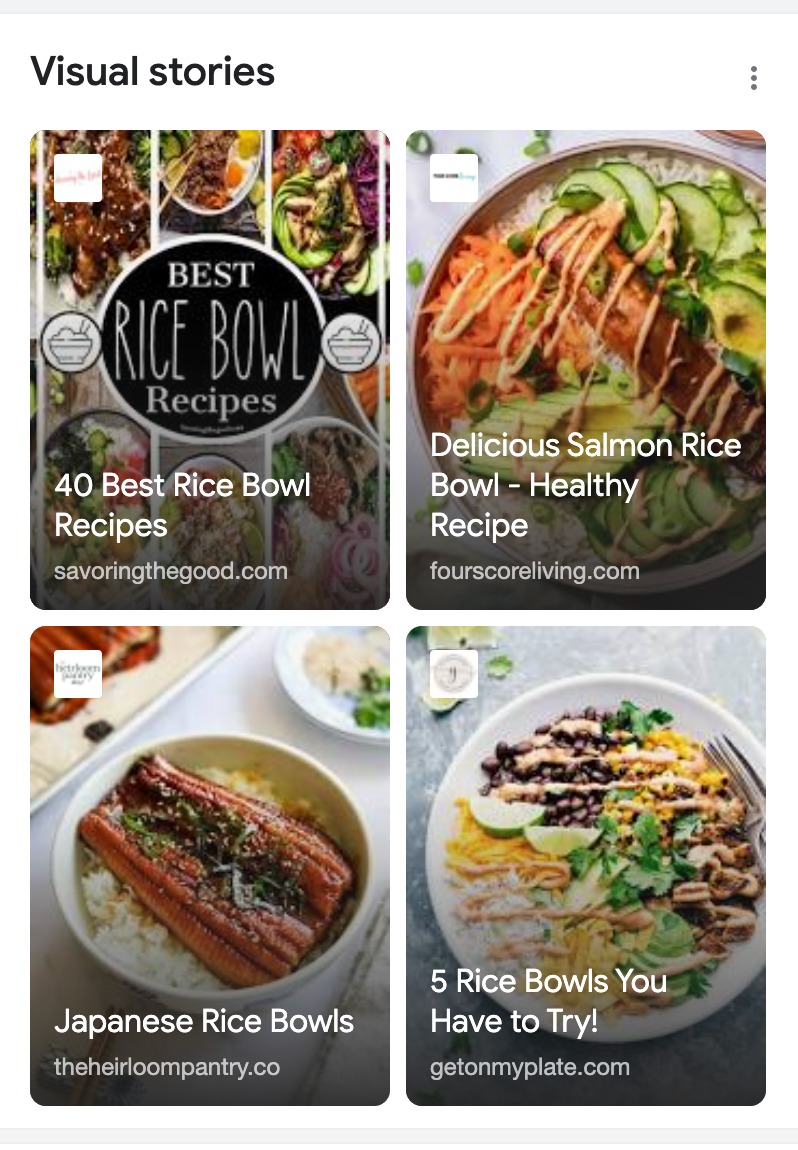This screenshot appears to be from a food-related section of a website, possibly resembling an Instagram-style platform due to its layout and presentation. The top-left corner of the screenshot features the text "Visual Stories" in black, indicating the themed content.

The screenshot showcases four different food stories, all centered around rice bowl recipes:

1. **Top-Left Thumbnail**: This section is titled "Best Rice Bowl Recipes" and links to an article titled "40 Best Rice Bowl Recipes" from savoringthegood.com. It is likely a comprehensive list of rice bowl recipes.

2. **Bottom-Left Thumbnail**: This story is labeled "Japanese Rice Bowls," featuring an image of a bowl with what looks like salmon and rice. The content originates from theheirloompantry.co, suggesting a focus on traditional or heritage-inspired Japanese rice bowls.

3. **Top-Right Thumbnail**: Displayed here is "Delicious Salmon Rice Bowl - Healthy Recipe," a recipe from fourscoreliving.com, showcasing a nutritious option among rice bowls.

4. **Bottom-Right Thumbnail**: This segment is titled "Five Rice Bowls You Have to Try," linking to an article from getonmyplate.com, promising a curated list of must-try rice bowl recipes.

The visual stories primarily reflect a user's apparent interest in rice bowl recipes, indicating they may have specifically searched for or shown a preference for this type of culinary content on the website.